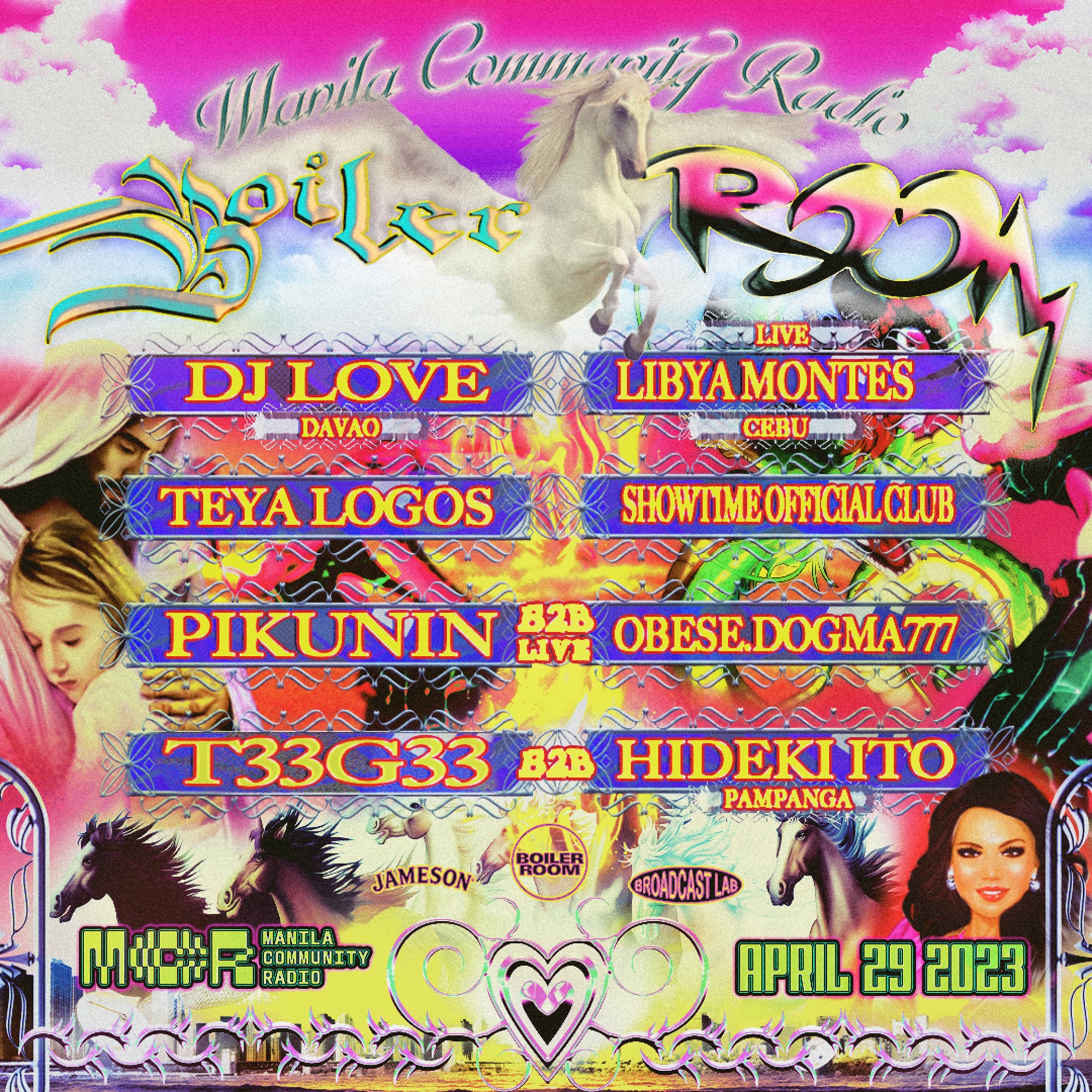This is a vibrant and busy promotional poster for Manila Community Radio's event on April 29, 2023. Dominated by an eye-catching purplish-pink gradient background with white clouds, the poster features an array of colorful details and hand-drawn elements. At the top, in a mix of cursive gray and white, the title "Manila Community Radio" stands out, followed by the words "Boiler Room" split between green and black-purple lettering, with a Pegasus flying between them.

The poster highlights a group of performing artists listed in yellow letters against a purple bar: DJ Love, Libia Montez, Taya Logo, Showtime Official Club, Pikunin, ObisDog, MA777, T33G33, and Hideki Ito. Illustrations on the poster include multiple horses, a central white horse, and pictures of a lady and a man in a shawl holding a little girl, contributing to its busy and colorful aesthetic.

Notably, the lower section of the poster includes a pink heart with floral details and chain-link flourishes framing the bottom border. The left corner features the Manila Community Radio logo, while the bottom right corner marks the event's date with additional sketches of a woman and a horse, enriching the overall artistic and dynamic design.